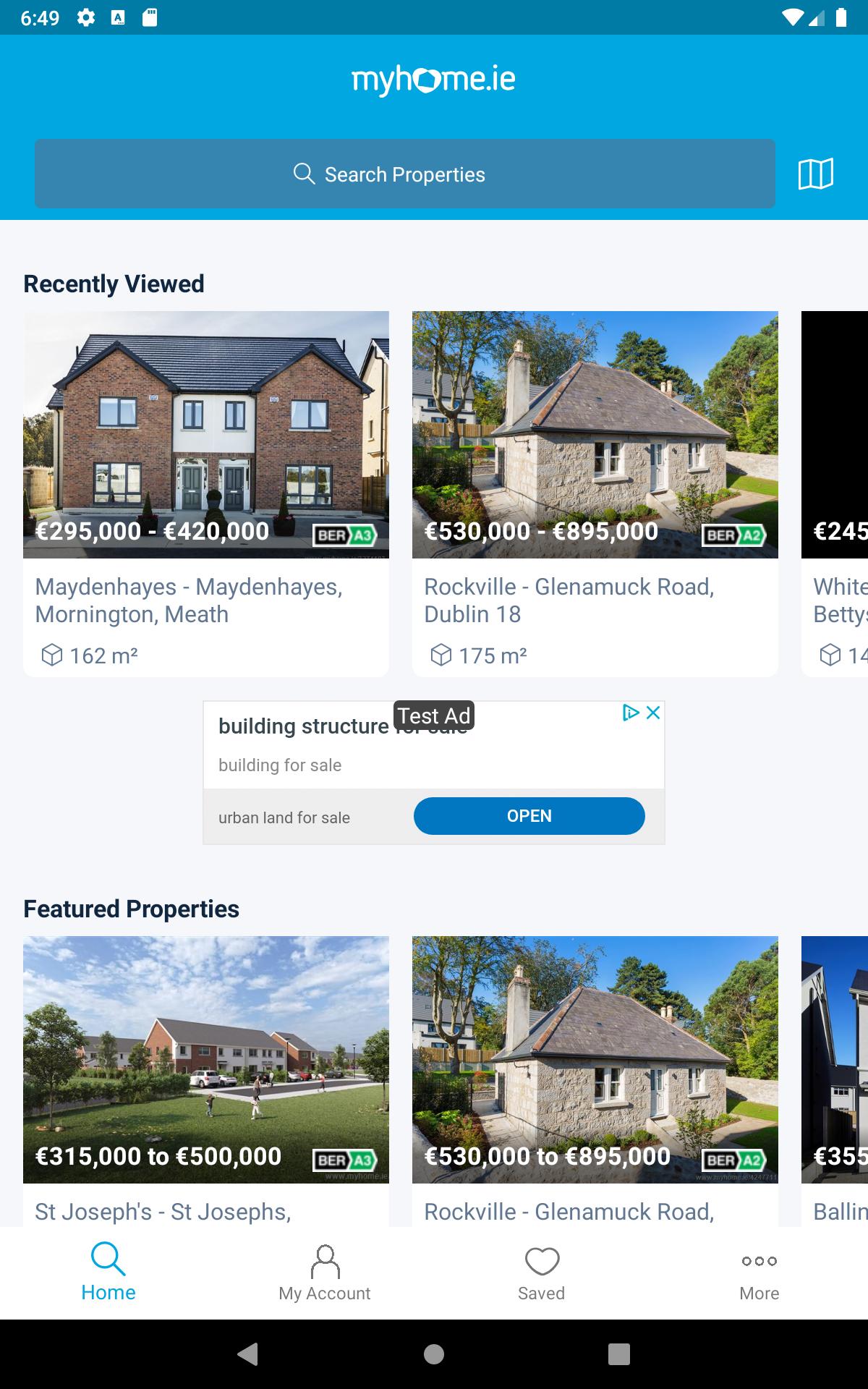A screenshot displays the homepage of the MyHome.ie mobile application on an Android device. Dominated by a blue color theme, the page features a prominent "Search Properties" banner alongside a search bar and a bookmark button. Beneath this, users can access their recently viewed properties. The main content showcases various homes, with a distinctive ad for building structures marked as a "Test Ad" appearing among the listings. Highlighted sections labeled "Featured Properties" present a curated list of notable listings. At the very bottom, navigation options such as "Home," "My Account," and "Save More" are visible, along with the Android navigation buttons. The status bar at the top left shows the current time, gear icon for settings, WiFi connectivity, and a fully charged battery. The interface is neatly organized, providing users with seamless property browsing capabilities.